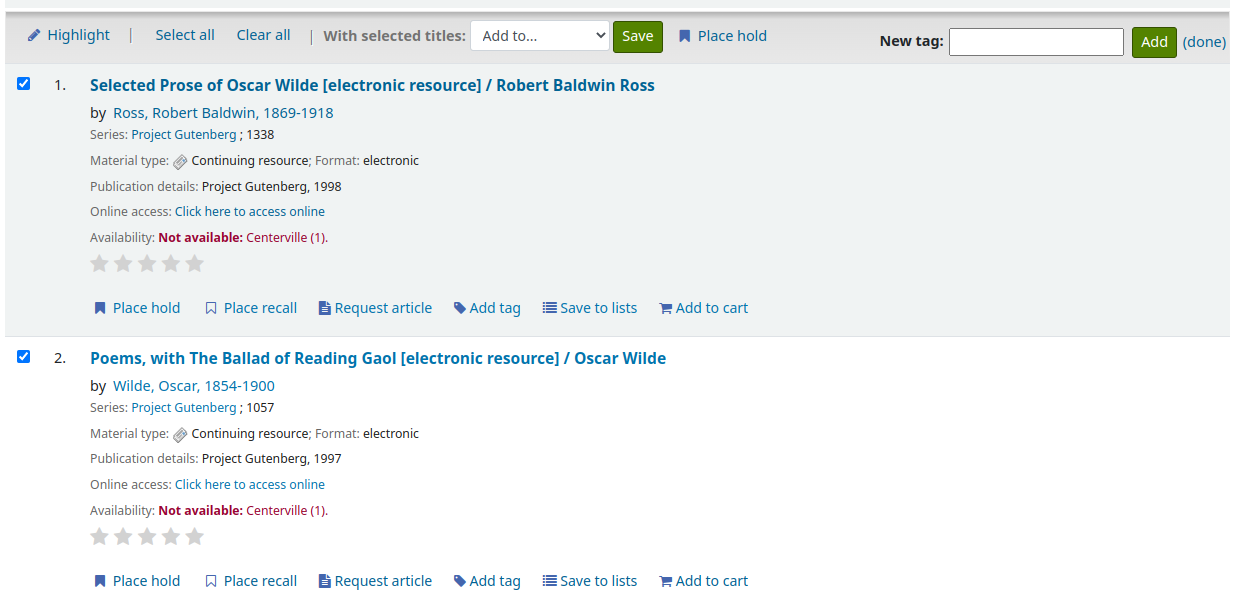Screenshot of a library search results page displaying two results. This page offers various options at the top, including buttons to highlight, select all, clear all, and a drop-down menu labeled "With selected titles," which includes options to add to, save, place hold, add new tag, and add. 

The search results are presented in a list format with a two-tone background where the top result has a gray background and the bottom result has a white background. 

1. **Selected Prose of Oscar Wilde** - This entry appears with a gray background and is listed as an electronic resource.
2. **Poems with The Ballad of Reading Gaol** - This entry appears with a white background and is also listed as an electronic resource.